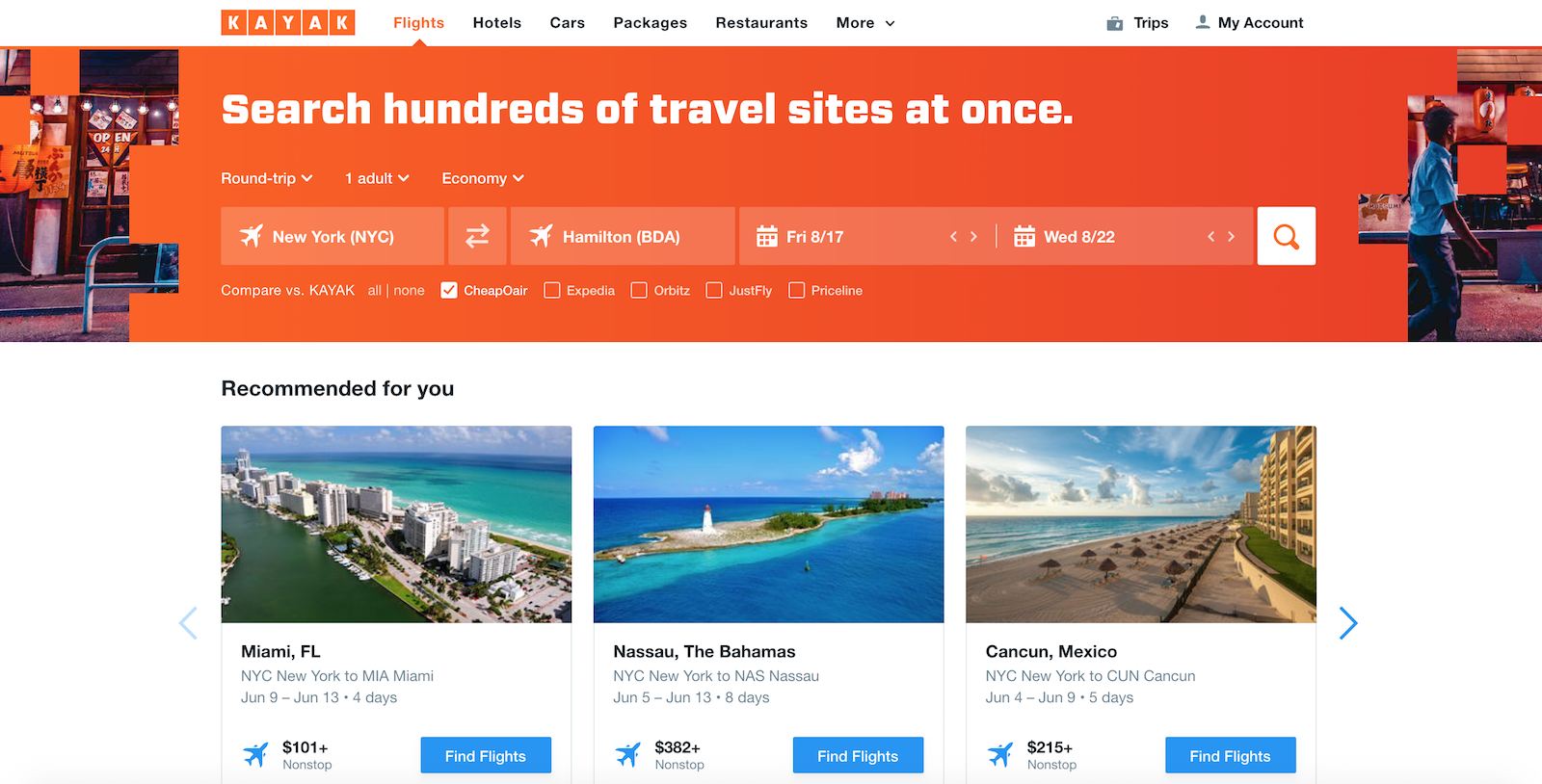A screenshot from a travel website prominently displays its user interface. At the top right corner, you find "My Account," and to its left, the word "Trips." On the top left, the word "KAYAK" appears in white text, each letter enclosed in an orange square. Next to this, a navigation menu features categories such as "Flights" (highlighted in orange), and "Hotels," "Cars," "Packages," "Restaurants," and "More" in black text.

Centered at the top middle section is the phrase "Search hundreds of travel sites at once." Below it is a series of boxed input areas for booking travel. The first box on the left displays "New York, NYC." Adjacent is a small box with arrows pointing left and right. The third box reads "Hamilton, BDA." Followed by two boxes showing date selections: "Friday, 8-17" and "8-22."

In the bottom half of the image, the text "Recommended for you" can be seen on the middle left, under which three boxed areas display destination suggestions: "Miami, Florida," "Nassau, The Bahamas," and "Cancun, Mexico." 

The layout and design elements suggest a user-friendly interface intended to streamline travel planning and bookings.